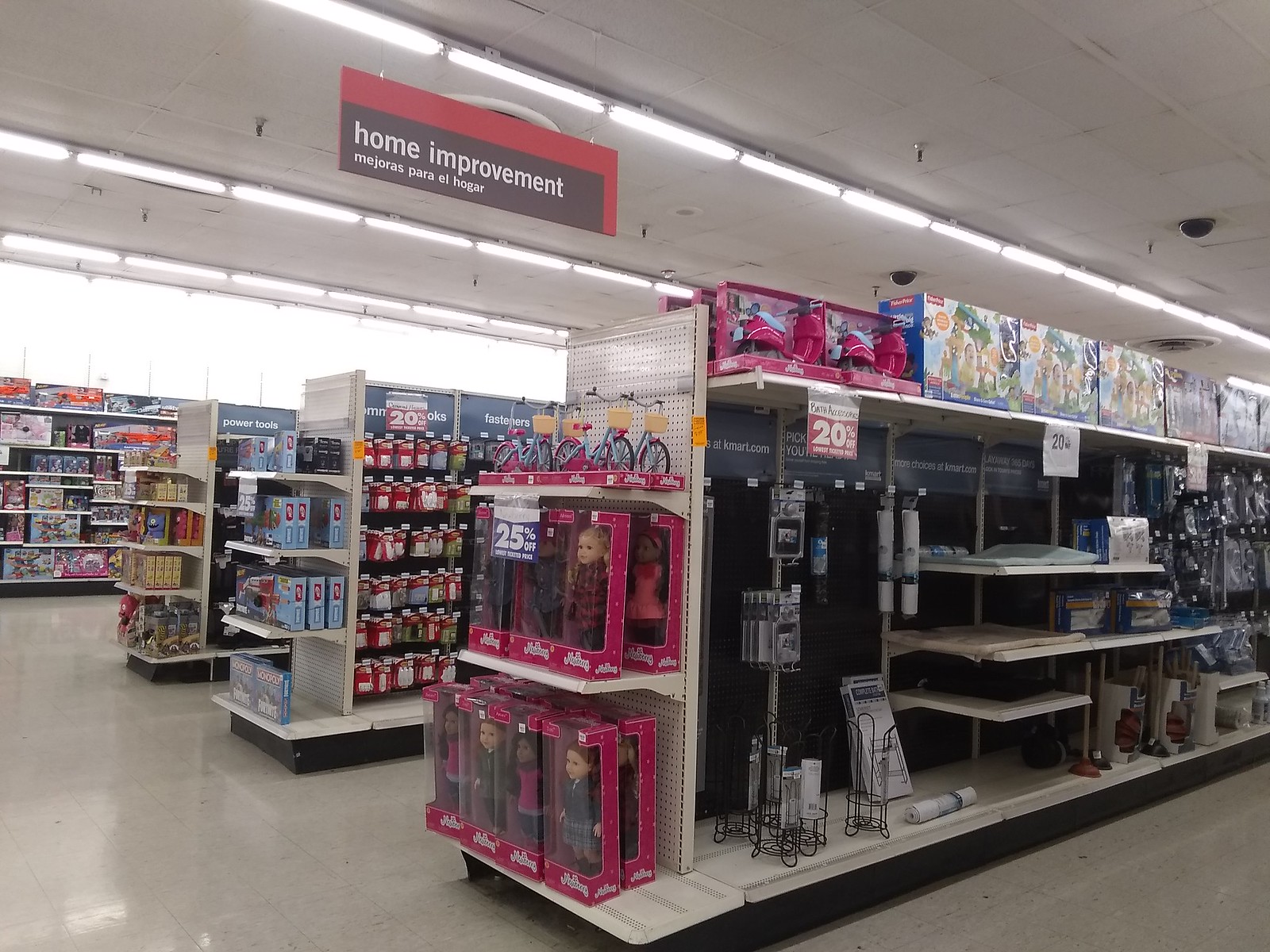In this bustling supermarket, three aisles stretch out, separated by dividers, with a wide view of meticulously arranged merchandise along the far wall to the left. In the foreground, an enticing display features boxes of dolls adorned with a "25% off" sign, prominently showcased with white text on a purple background. The pink doll boxes, approximately two feet in length, have clear plastic windows revealing the dolls within. To the right, additional shelves host various housewares, though some are partially empty. Bright "20% off" signs are interspersed among the items, signaling numerous discounts throughout this vibrant retail space.